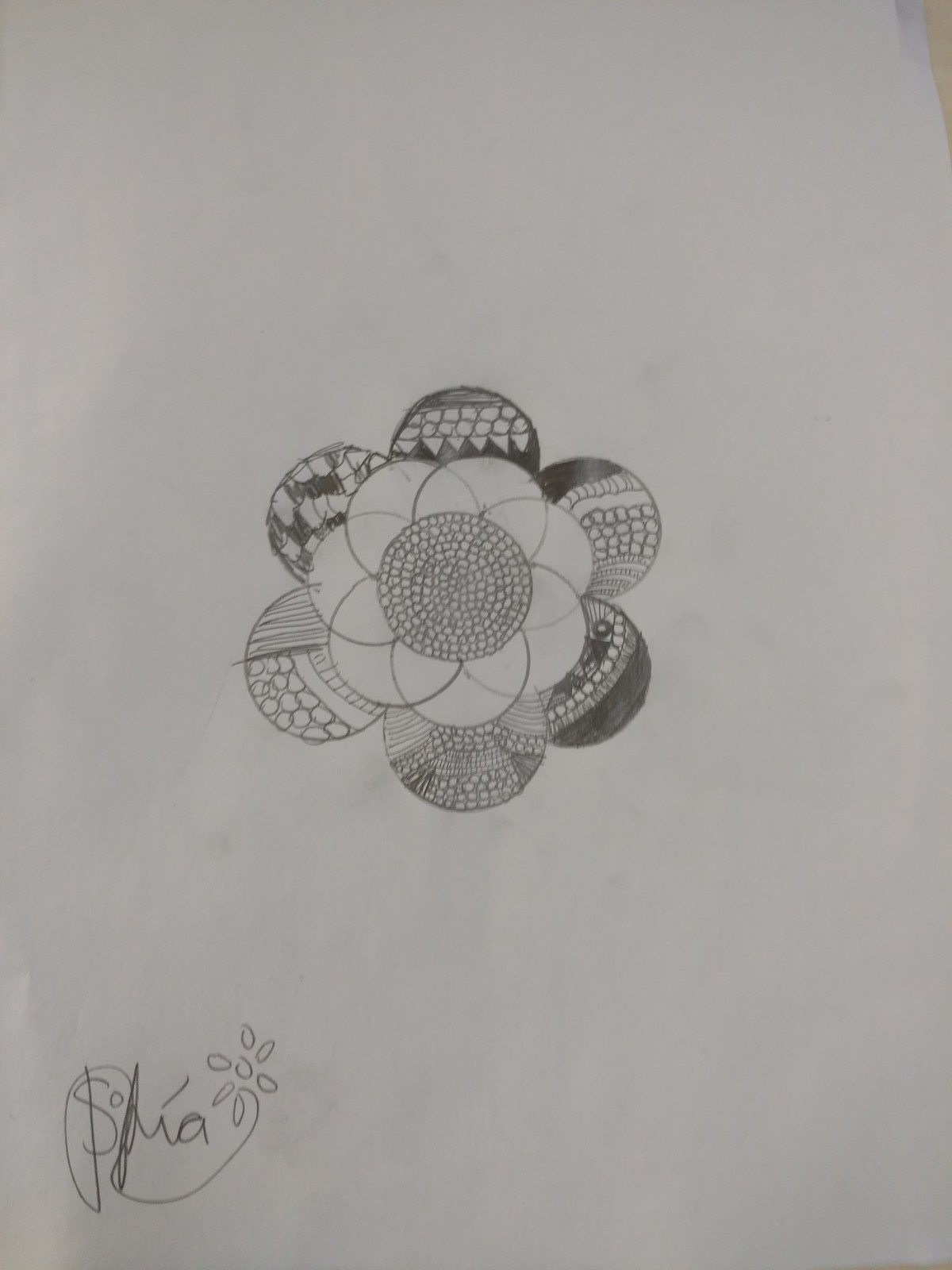This is a close-up photograph of a geometric drawing of a stylized flower on a white piece of paper. The paper exhibits some black smudges, likely from the pencil used, and has visible creases on the lower left side. The artist’s signature, which appears to be "S-H-M-A" with an accent over the 'M' and an elaborate swirl through the 'S' and 'M,' is also located on the lower left. This signature intricately connects to a flower-like symbol consisting of interconnected circles and ovals.

At the core of the drawing, small interconnected circles form a central circle. This is encircled by slightly larger circles that interlink with both the central circle and each other, creating petal-like shapes. Beyond this, a third layer of circles overlaps the second, extending the floral design. Each of the six outer petals displays unique patterns including various configurations of lines, circles, triangles, and trapezoids in shades of black and gray. 

The top petal features alternating horizontal dark gray lines, white circles, and interlocking triangles of contrasting colors. Others include designs such as lines with circles, unfilled circles, dark triangles, hash marks, and mixed trapezoidal shapes in black, white, and gray. The drawing’s precise, geometric style and detailed texturing suggest a sophisticated representation of a flower, with elements that might also evoke the structural variety of soil.